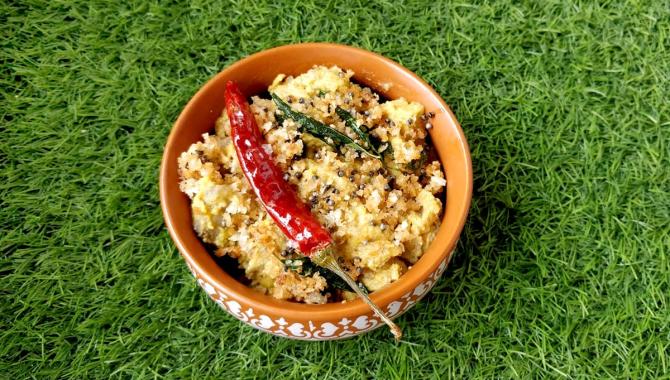This vibrant photo captures a bird’s-eye view of an ornate orange ceramic bowl with a delicate white pattern on its exterior, set against a vivid, well-manicured green grass backdrop. The bowl is overflowing with a mixture that appears to be light yellow-orange quinoa or a similar seed-based dish. Prominently displayed on top is a long, skinny red chili pepper, accompanied by what seems to be green leafy vegetables, possibly spinach. The image, devoid of text, evokes the aesthetic of food photography typically seen in culinary magazines, focusing on the contrasting colors and textures of the ingredients and their picturesque presentation on the lush grass.